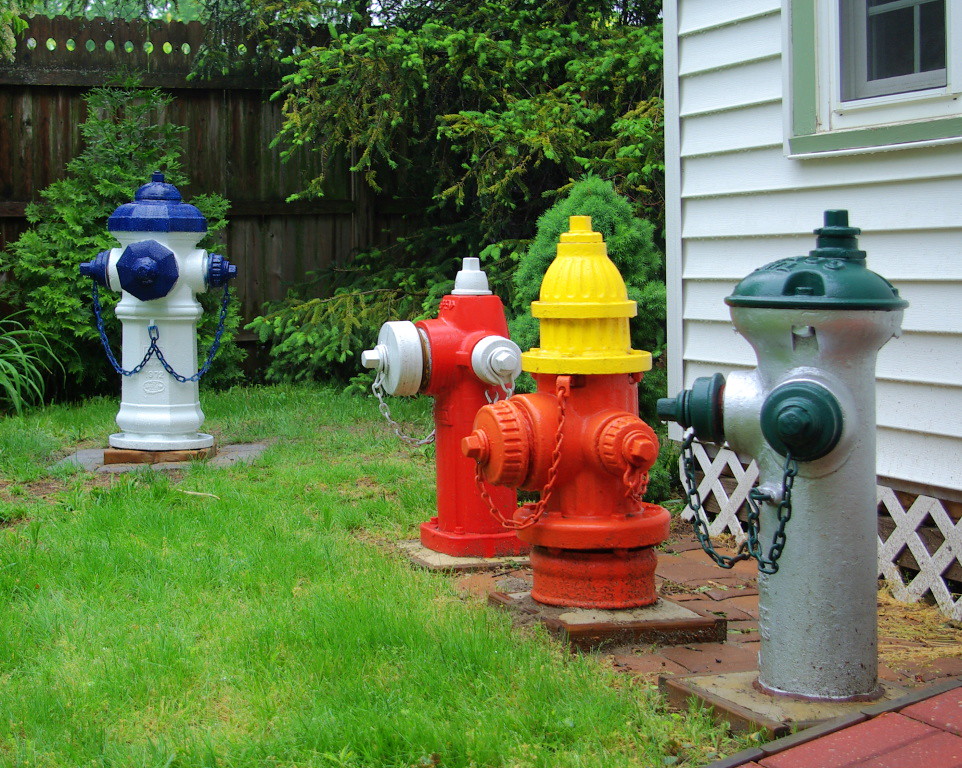This vivid color photograph depicts a backyard scene showcasing a unique collection of four multicolored fire hydrants, meticulously arranged on a bright green lawn. On the left side, set slightly apart, is a fire hydrant painted white with blue spouts and a matching blue chain. Central to the image, a red hydrant with white accents stands beside another red hydrant featuring a yellow top. The far right presents a silver hydrant adorned with green accents and a coordinating green chain. Behind this eclectic lineup, a white wooden house with a plank-style wall and a light sage green window border is partly visible. The bottom right corner reveals a segment of a red brick pathway. On the upper left, a dark brown wooden fence encloses lush green trees and shrubs, completing the picturesque scene.